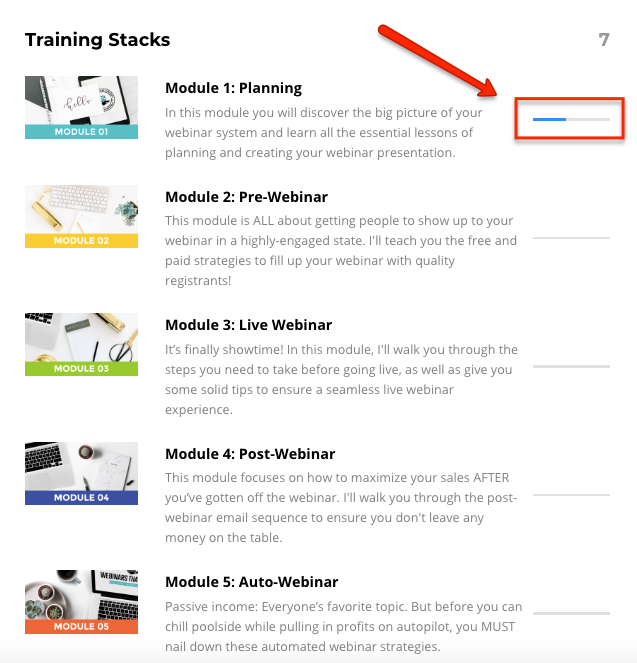**Detailed Caption:**

In the upper left-hand corner of the image, there is a detailed training stack consisting of five vertically aligned modules, each thoughtfully designed to guide users through the process of planning and executing webinars. The stack is visually organized with each module labeled clearly:

1. **Module 1: Planning**
   - This introductory module focuses on the foundational aspects of webinar planning. It promises to equip participants with a comprehensive understanding of the webinar system, covering all essential lessons on planning and creating effective webinar presentations.
   - A prominent progress bar located to the right of this module indicates the user's completion status. This bar is encased in a red, square outline reminiscent of a Photoshop design element, and is nearly halfway filled. A red arrow sharply points towards the progress bar, drawing attention to the user's current advancement.

2. **Module 2: Pre-Webinar**
   - This module covers all the preparatory actions required before the live event, ensuring that participants are well-prepared and ready to engage their audience.

3. **Module 3: Live Webinar**
   - Marked with the phrase "It's finally showtime," this module guides participants through the critical steps necessary for hosting a live webinar. Detailed instructions help users gain confidence and manage the live event seamlessly.

4. **Module 4: Post-Webinar**
   - This module provides strategies and steps to follow after the webinar concludes, emphasizing follow-up actions and participant engagement to maximize the event's impact.

5. **Module 5: Auto-Webinar**
   - Focused on the concept of "passive income," this module teaches participants how to set up automated webinars. This is presented as a favorite topic, likely because of its promise of ongoing benefits with minimized effort.

Overall, the image offers a well-organized, step-by-step training approach tailored for webinar success, visually enhanced with progress indicators and attention-drawing elements.